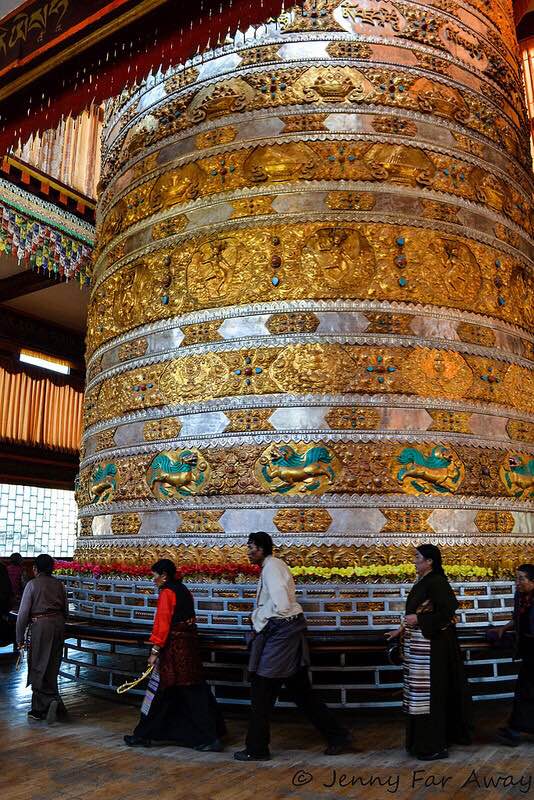This color photograph by Jenny Faraway captures an intricate and ornately designed pillar inside what appears to be a temple or a similarly significant cultural building, likely in Eastern Asia. The central pillar, which extends impressively from the floor to the ceiling, is adorned with alternating silver and gold stripes, each detailed with geometric shapes, embossed figures, and stylized lions or dragons. Notable are the lions with turquoise manes and gold lion faces accented with turquoise elements. The pillar features numerous small, embedded red and blue gems, contributing to its intricate beauty. In the photograph, several individuals, including men and women wearing traditional Indian clothing, walk in single file around the pillar on a worn path, suggesting a form of worship or ritual. A man in a black outfit with a striped apron also features among the people. The floor and surrounding area are richly detailed, and a small fence seems to prevent people from getting too close to the pillar. The caption "Copyright Jenny Faraway" is visible in the bottom right corner of the image.